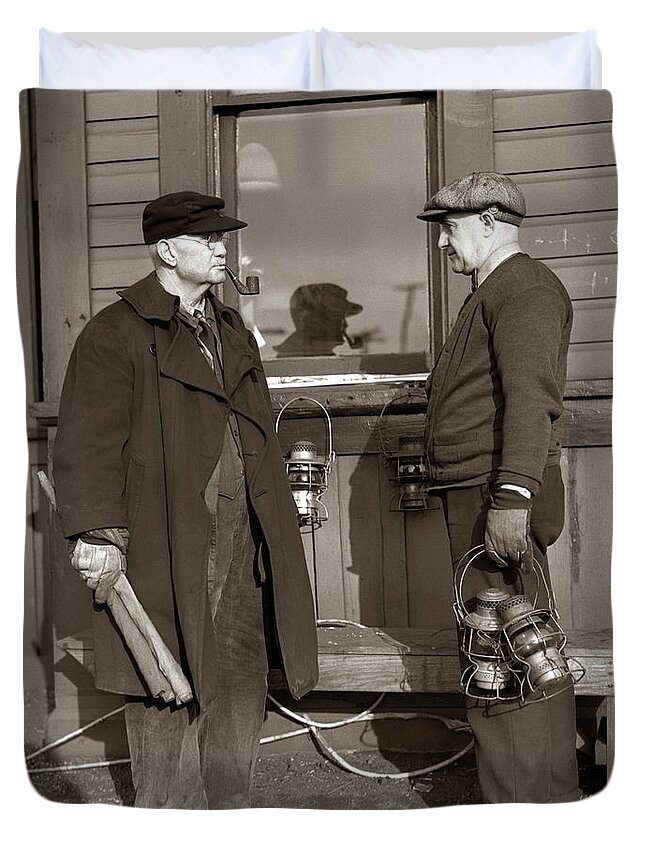In this detailed depiction, a digitally cropped, aged black-and-white photograph, likely tinted into a dark sepia tone, portrays two older white males, seemingly in their 50s or 60s, standing face-to-face in front of a wooden house during daylight. The photograph itself is portrait-oriented with irregular, somewhat lumpy edges, suggesting it was manually edited. A pair of white cloth curtains peeks out from above the image, partially obscured behind the photograph.

The backdrop includes a glass window on the wooden house, reflecting the man on the left. Between the men, two lanterns are nailed to the house at slightly above waist height. On the ground, resembling a dirt surface, various wires are scattered.

The man on the right is dressed in a hat, a sweater cardigan, long pants, and gloves. His hat is a grayish tabby tone, and he holds two silver lanterns in his gloved hand, staring neutrally at the man on the left. The man on the left, also gazing neutrally back, features round glasses and a pipe protruding from his mouth beneath a flat-brimmed black hat. He dons a long black coat, possibly covering denim work overalls or lighter-colored pants. In his right hand, he holds what appears to be two rolled-up pieces of paper or torches. Both men are bathed in sunlight, casting distinct shadows on the house behind them.